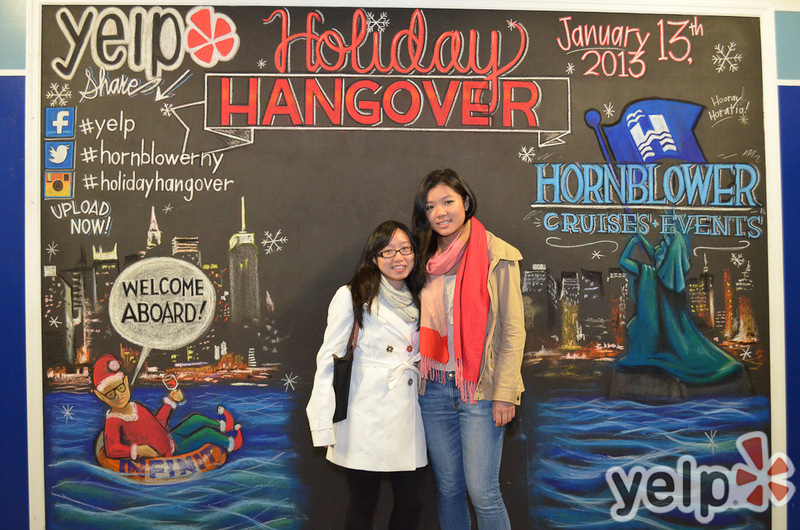This full-color photograph features two young Asian women standing side by side and posing for the camera. The shorter of the two, on the left, has long dark hair, wears dark-framed glasses, a white jacket, black pants, and carries a black bag over her shoulder. The taller woman on the right also has long dark hair and is dressed in a tan jacket paired with a red and pink scarf, a white shirt, and light blue jeans. Both women are smiling warmly at the camera.

The backdrop behind them is predominantly black with red text at the top reading "Holiday Hangover" and is adorned with various logos and hashtags: "Yelp," "#HornblowerNY," and "#HolidayHangover" for Facebook, Twitter, and Instagram respectively. 

The scene behind them depicts a whimsical chalk drawing of a nighttime cityscape by a river. There is blue water with a Christmas elf, dressed in traditional festive attire, floating on an inner tube while holding a flag and cheerfully greeting with "Welcome Aboard." To the right of the elf stands a statue of a lady blowing a horn, labeled "Hornblower Cruises and Events." The date "January 13th, 2003" is also visible among the backdrop elements.